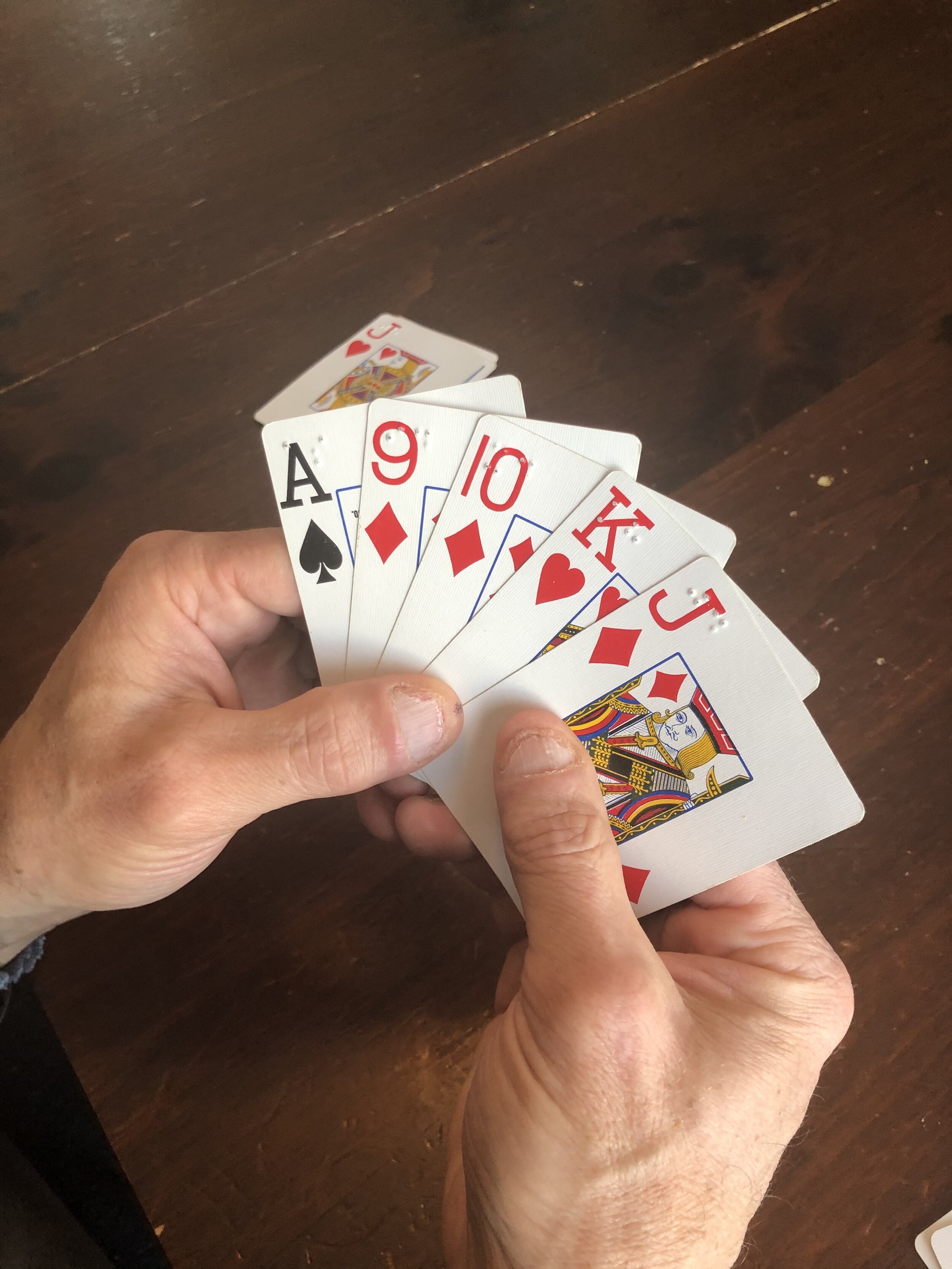The image showcases a close-up, top-down view of a white-skinned man's hands, with chewed down nails, holding a hand of playing cards. His hands emerge from the lower left corner of the photograph, gripping the cards between his thumbs and index fingers. The cards displayed are an Ace of Spades, a Nine of Diamonds, a Ten of Diamonds, a King of Hearts, and a Jack of Diamonds, each featuring larger-than-usual numbers and letters along with Braille in the upper left corner for accessibility. The cards have a white background with traditional illustrations, including a royal-looking Jack of Diamonds. On the wooden, sectioned table with a visible wood grain, there is a Jack of Hearts card laying face up, also in larger, easy-to-read print. The focused and zoomed-in nature of the photo does not reveal any additional players or the full table, emphasizing the solitary scene and detailed depiction of the cards and hands.